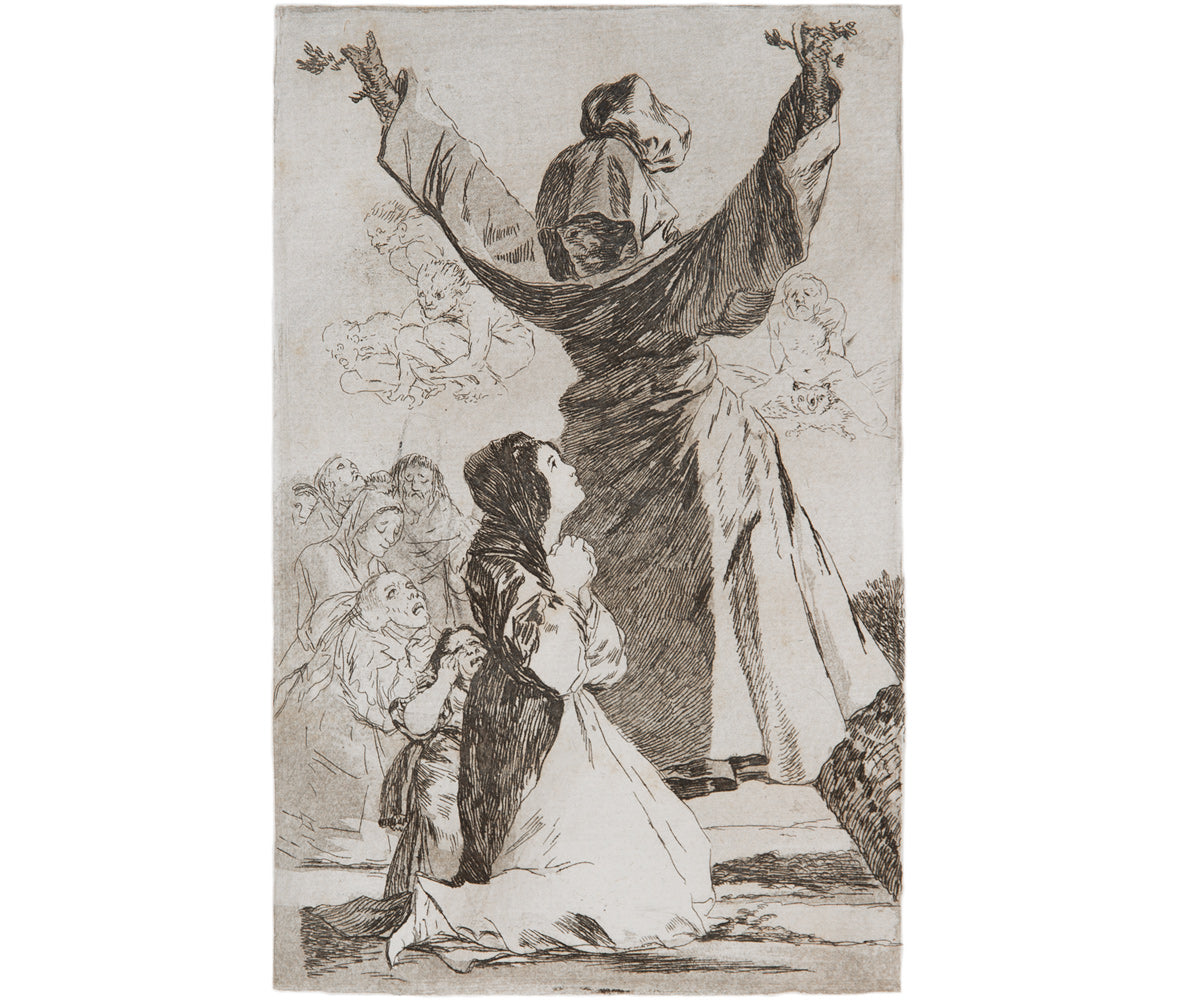This detailed black and white line drawing appears as an ink illustration capturing a surreal, almost nightmarish scene. At the center stands a towering, hooded figure draped in a robe-like gown. Its knobby, gnarled hands, resembling twisted tree branches, are outstretched in a menacing or commanding gesture. The figure's face is shadowed under the hood, adding to its ominous presence. Kneeling before this looming entity is a woman in a white dress, her hands clasped in prayer or supplication. She is also cloaked in a dark shawl extending past her gown. Behind her, another woman with short brown hair, also clad in white, watches the scene unfold. To the right of this central tableau, a bent-over winged man adds to the eerie atmosphere. The background is populated by faintly drawn figures of people and small, goblin-like creatures, all seemingly in awe or fear of the giant figure. The scene is otherworldly, invoking a sense of dread and reverence, with the kneeling individuals and the hooded giant forming the focal points of this unsettling artwork.